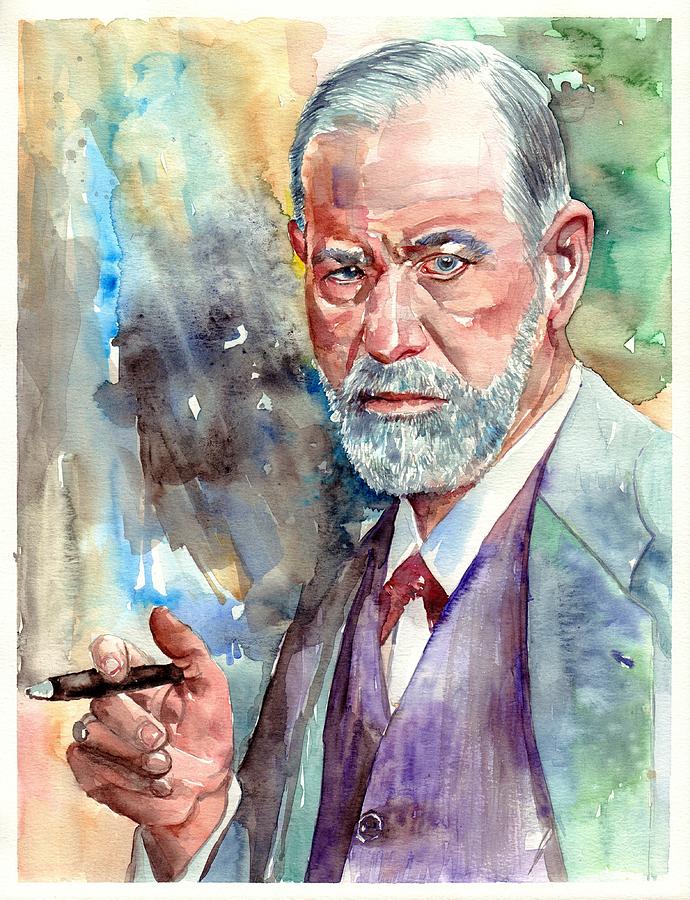The image is a watercolor painting of a Caucasian white gentleman, estimated to be between his mid-60s and early 70s. The composition captures the man's head, part of his shoulders, and his right hand, which holds a small brown cigar with slightly dirty nails, adorned by a ring on his finger. The gentleman has gray and white hair, tidily parted and combed, and a full beard and mustache that exhibit shades of brown and gray. His eyes are blue, conveying a pensive, almost concerned expression.

His attire includes a green jacket with various pastel shades, a purple vest, and a white collared shirt. At his neck, he wears a red cravat that is neither a typical bow tie nor a standard tie, adding an unusual touch to his distinguished appearance. The background is an abstract mix of pastel colors including green, sandy tones, blue, and purple, enhancing the gentleman's prominent, almost photorealistic presence. The overall mood and finely captured light and shadow contribute to a professorial and contemplative aura, making him the undeniable focal point of the painting.